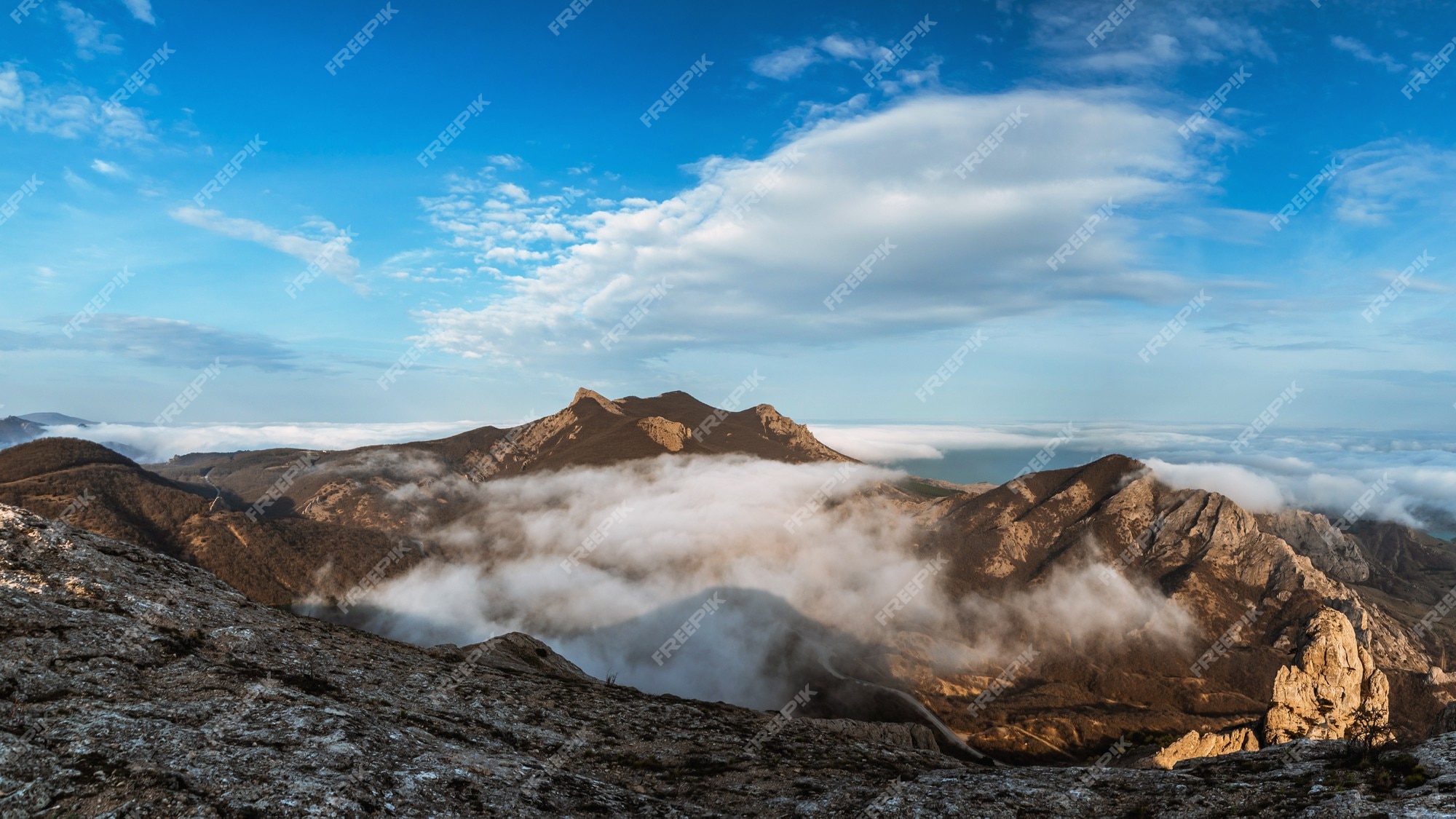The photograph showcases a breathtaking mountain scene captured from a high vantage point, possibly the peak of a mountain range. The foreground features a rugged mountain top with visible details of rocks, dirt, and sparse vegetation. The expansive view reveals a series of mountain peaks stretching into the distance, characterized by brown, rocky faces and patches of tree cover. Fluffy white clouds float around and just above the mountains, blending into a mostly clear, pastel blue sky. The serene natural beauty is slightly marred by the presence of multiple "Freepik" watermarks, printed in white and angled diagonally across the image, indicating the photo's copyrighted status. The contrast of the earthy mountain tones with the bright sky and clouds creates a striking visual.